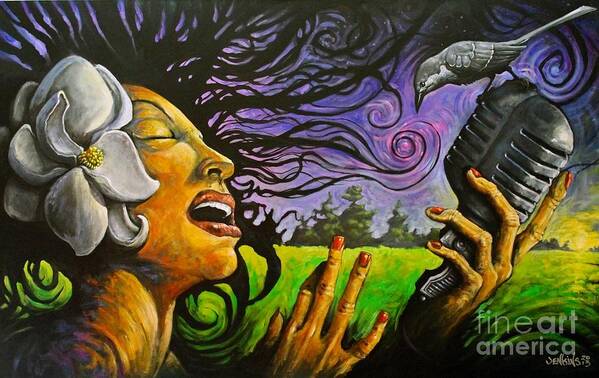This detailed illustrated image resembles a painting and features a captivating scene of a woman deeply immersed in singing. She is positioned to the left of the frame, facing right, and holds an antique silver microphone, to which a small grayish-black bird perches, facing her. Her expressive posture, with one hand grasping the microphone and the other raised with spread fingers, conveys her profound connection to her music. The woman’s face is slightly upturned, her eyes closed, and her mouth open, evoking a deep emotional engagement with her performance. Her dark brown hair, adorned with a large white flower, swirls and twirls in all directions, seamlessly blending with a Van Gogh-esque Starry Night sky filled with bluish-purple tones. The scene is set against a backdrop of a green field and distant trees. Her long, slender fingers with red nails add to the elegance of the image. At the bottom right, a watermark says "Fine Art America," and just below it, the signature "Jenkins" is faintly discernible, possibly marking the year "95."